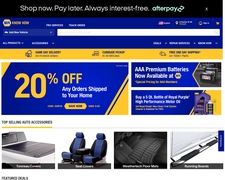The image depicts a sales flyer webpage from Napa Auto Parts. At the top of the screen, a black banner with white text invites customers to "Shop now, Pay later, Always interest-free." Accompanying this message is the Afterpay logo in a light aqua green color. Directly below this banner is a title bar featuring the word "Napa" prominently displayed in white font against a royal blue background. Adjacent to the title is a white search bar designed for users to look up specific items.

Beneath the royal blue section is a yellowish-orange bar highlighted with royal blue text. This section provides information on three distinct features or announcements. Further down, the webpage showcases ongoing promotions. One notable promotion offers 20% off on any orders shipped to home addresses, while another highlights AAA premium batteries. Below these promotional banners, there is a display of various products available for purchase.